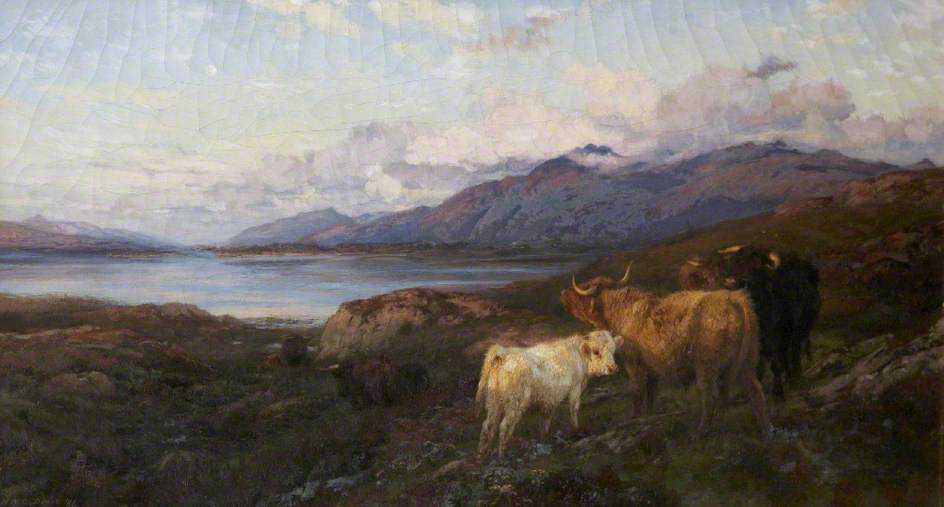This detailed painting, likely executed in watercolors, depicts a serene countryside landscape featuring several animals. In the background, white and gray fluffy clouds drift above a small, hill-like mountainous form, emphasizing the distant horizon's tranquility. Below the hills lies a calm body of water, possibly a pond or lake, that reflects the serene sky above. The landscape is punctuated by rocky formations. To the bottom right of the painting, three distinct cows are prominently featured. The smallest is a white calf, standing nearest to us with its rear slightly angled toward the viewer. Next to the calf, a light tan cow with small yet prominent horns gazes towards the sky or sunset, adding a sense of calm contemplation. Beside this horned cow stands a darker, muddied brown cow, blending into the pastoral scene. The entire artwork hints at age, as the top of the painting appears cracked, possibly suggesting that the piece has weathered time, adding to its rustic charm.